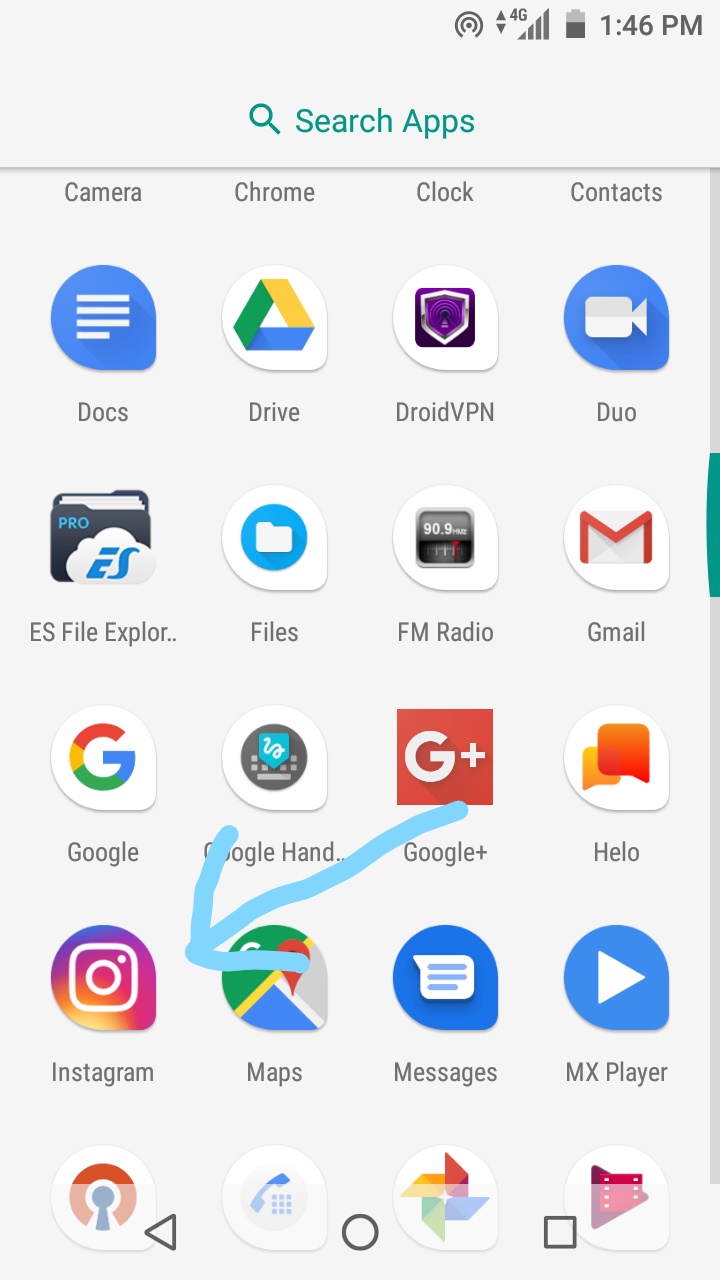The image shows the app drawer of an Android phone, featuring a variety of application icons. While not all app names are visible, clearly identifiable ones include Docs, Drive, Camera, Chrome, Cloud Contacts (without icons), DroidVPN, Duo, ES File Explorer, Files, FM Radio, Gmail, Google (something), Google Plus, and one with hand gestures. Other visible icons include Hello, 1L, Instagram, Maps, Messages, and App Explorer. Some app names are truncated, but discernible ones likely include Photos and Play Movies. 

An arrow, seemingly drawn in light blue and somewhat crudely added, points to the Instagram icon. This arrow has a teardrop shape, tapering towards the bottom right. While many icons follow this teardrop format, some seem irregular and do not conform to this shape.